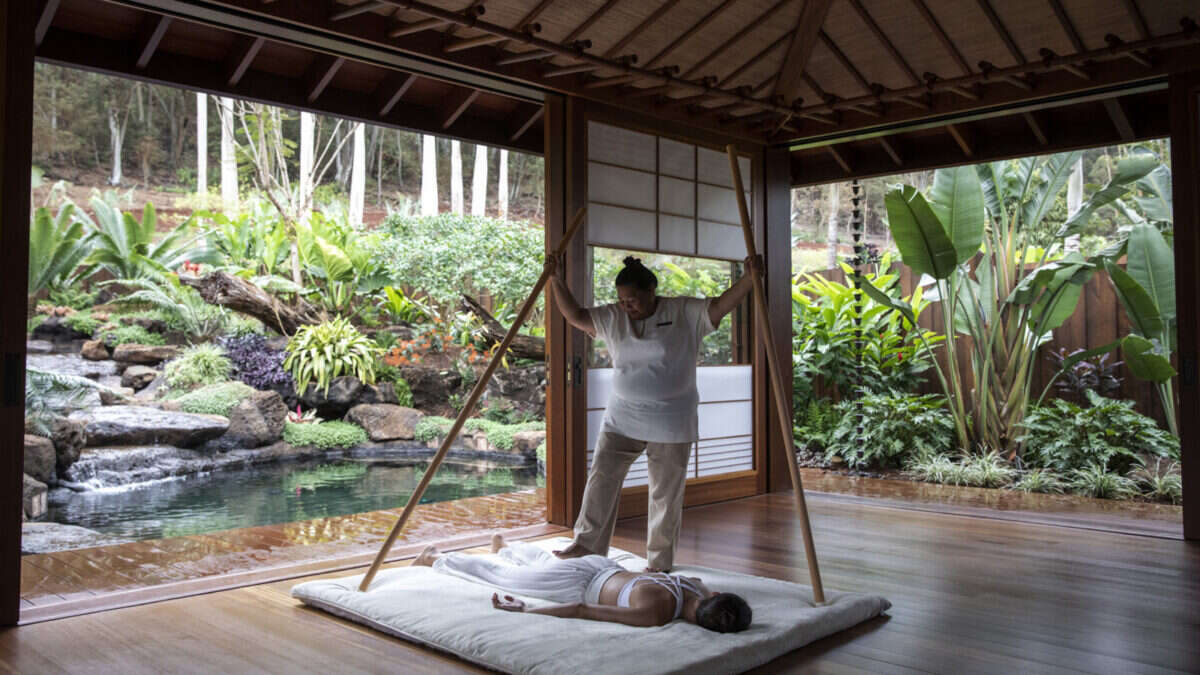In the image, a serene Japanese-style pagoda serves as the backdrop, featuring traditional architecture with rich redwood elements and white paper walls adorned with wooden grids. The building's open sliding paper doors reveal a lush, meticulously maintained garden outside, complete with diverse trees, foliage, a rock garden, and a serene pond.

Inside, both the polished, highly reflective wooden floor and the overall environment exude cleanliness. At the center of this tranquil setting, a woman wearing white silk pants and a white sports bra lies face down on a white mattress. Above her stands another woman, seemingly performing an orthopedic or therapeutic treatment. This practitioner, dressed in white pants and a white shirt, uses two tall brown sticks for support. One foot is placed cautiously on the patient's left buttock, suggesting she may be preparing to apply a form of pressure-based therapy, possibly a specialized massage technique.

The harmonious blend of the indoor pagoda aesthetics and the vibrant outdoor garden creates a peaceful ambiance, ideal for such a healing practice.